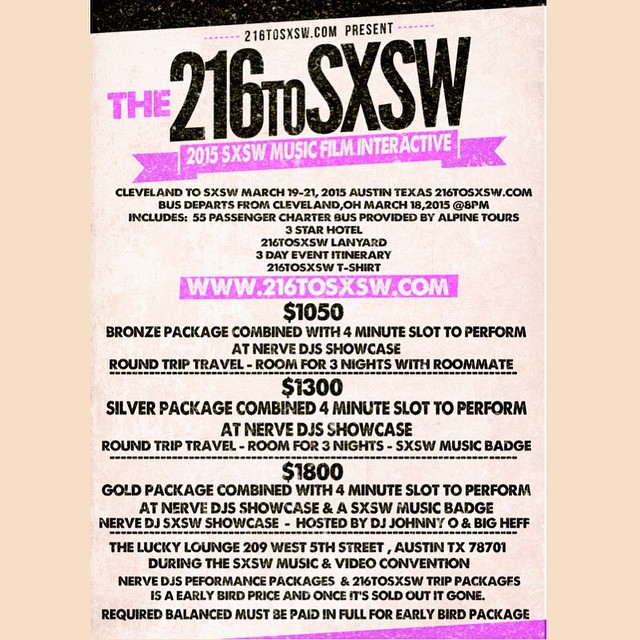The image is an advertisement for an event titled "216 to SXSW," which is headlined in a bold sans-serif black font. The flyer features a white background with a peach-colored border on both the left and right sides. At the top center, "216-SXSW.com" is prominently displayed. Below this header, it reads "Present the 216 to SXSW," followed by "2015 SXSW Music Film Interactive" in a mix of black and white text set against a purple ribbon.

The advertisement provides detailed package options for the event:

- **Bronze Package ($1,050)**: Includes specific benefits not entirely detailed in the description but positioned at the top of the pricing section.
- **Silver Package ($1,300)**: Offers a four-minute slot to perform, likely at the same venue and event as other packages, detailed beneath the bronze tier.
- **Gold Package ($1,800)**: Also includes a four-minute slot to perform at the Nerve DJ Showcase at SXSW Music Batch. This package is highlighted as the premium option.

Further down, in smaller black text against a gradient light pink background that darkens slightly on the right, additional event details are provided. The advertisement closes with the venue information: "The Lucky Lounge, 209 West 5th Street, Austin, TX."

The web address "www.216-SXSW.com" appears prominently again within a purple rectangle, ensuring potential attendees know where to find more information. Decorative elements include inclined black and purple borders that subtly angle to match the inclinations of the main header, adding a cohesive aesthetic flair to the overall design.